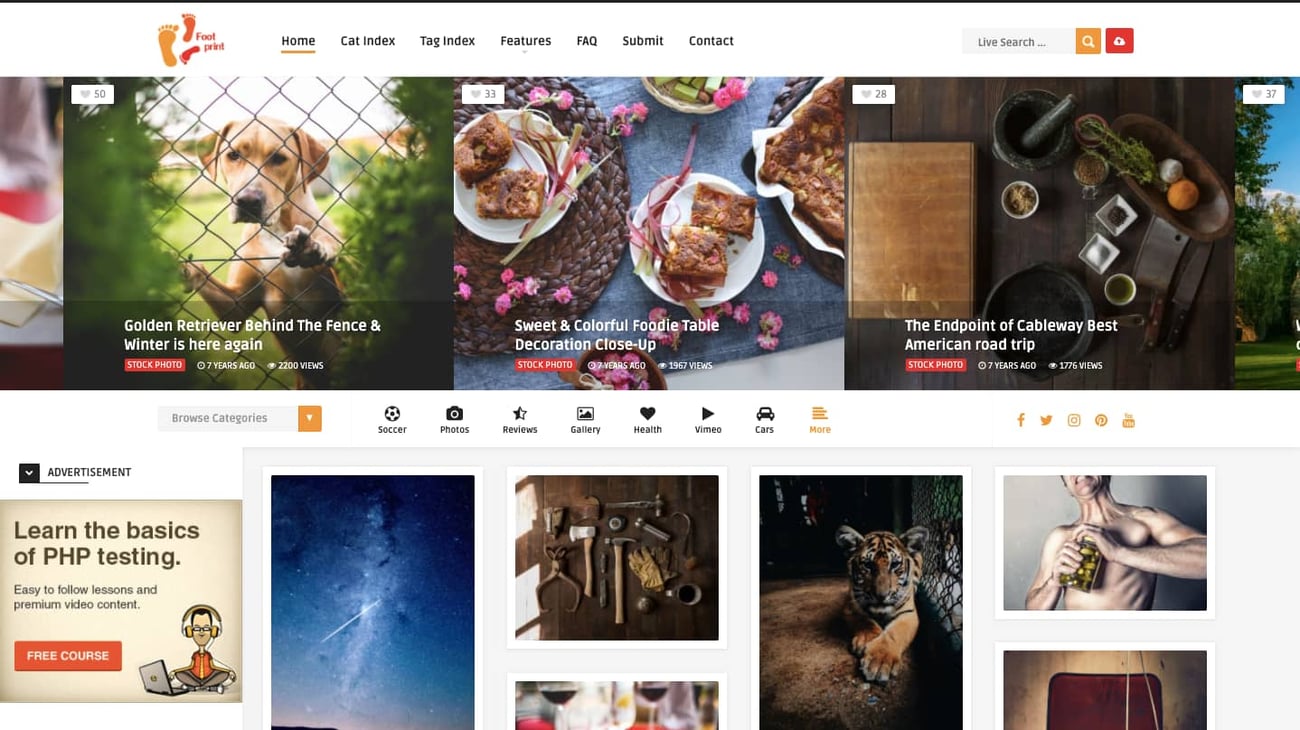This screenshot captures a webpage from the website Footprint. The logo, featuring an orange, a red, and a yellow foot forming a triangle, is prominently placed in the upper left corner. To the right of the logo, the word "Footprint" is displayed in a reddish font. The navigation menu at the top includes several tabs: Home (highlighted in yellow, indicating it is the current selection), Cat Index, Tag Index, Features, FAQ, Submit, and Contact. These tabs are in black font against a white background.

In the upper-right corner, there is a live search bar with a yellow magnifying glass icon for searching the site. Next to the search bar, there is a red button with a cloud and arrow icon, suggesting users can click to upload content.

Presently, the top section of the webpage features three main articles. The first article, titled "Golden Retriever Behind the Fence and Winter is Here Again," showcases an image of a Golden Retriever peeking through a chain-link fence. The second article, "Sweet and Colorful Foodie Table Decoration Close-ups," presents a close-up view of a beautifully decorated dessert table adorned with vibrant flowers. The third article, titled "The Endpoint of Cableway: Best American Road Trip," displays a rustic table setting with an old medicine bottle, antique knives, and various herbs.

Below these main articles, there are several other miscellaneous photos that users can click on for additional information.